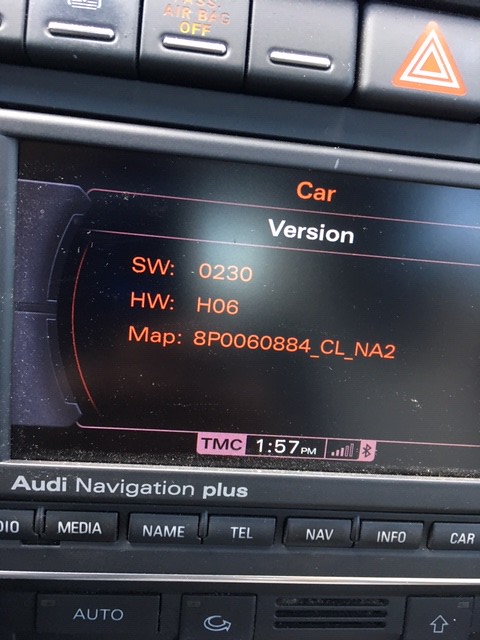The image showcases the dashboard of an Audi vehicle, specifically focusing on the car's stereo and control interface. The central element is a black screen displaying the text "car version" in orange and white fonts, followed by detailed version information: SW:0230, HW:H06, MAP:8P0060884__CL__NA2. Below this, a light pink banner provides additional information: "TMC" in black, the time "1:57 PM" in white, and a Bluetooth signal indicator with three out of five bars filled. The screen is flanked by various control buttons; above it are four buttons, including the "passenger airbag off" marked in orange and the "emergency flasher" with a triangle icon featuring smaller alternating color triangles. Located just below the screen, "Audi Navigation Plus" is prominently displayed. Beneath this inscription are seven white-labeled buttons for radio, media, name, telephone, navigation, information, and car functions. Further down, three more buttons are visible: "auto," a right-pointing arrow, and another arrow pointing upwards, next to a vent with three slats. The dashboard, a mix of charcoal gray and black, comprises a typical layout that Audi owners might recognize.